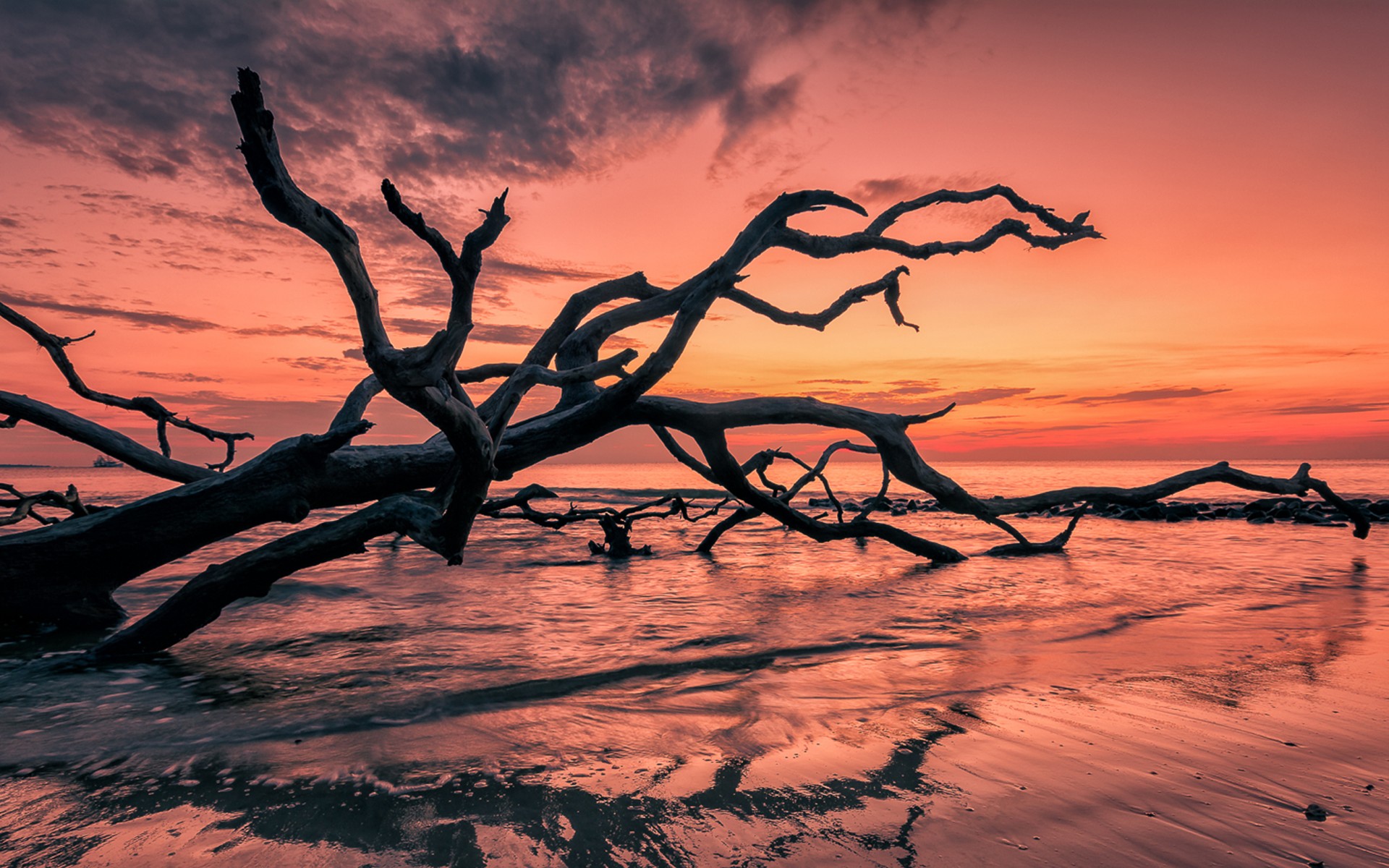The color photograph captures a mesmerizing sunset scene at the edge of the ocean, where a large, bare, dead tree—resembling driftwood—stands partially upright and partially fallen into the shallow water. Spanning from the left to the right side of the rectangular frame, the tree's dark and gnarled branches stretch out, devoid of any bark or leaves, giving a ghostly appearance. The sandy beach in the foreground is tinged with reflective hues of pink and orange from the breathtaking sunset, which dominates the upper part of the photo. The sky transitions from a deep amber at the horizon to softer pastels, interspersed with scattered spots of dark gray clouds. On the right-hand side, part of a rock jetty can be seen. The leaning driftwood tree forms a subtle arch over the water, beneath which a smaller branch rests atop some rocks. The beach appears shiny from the constant ebb and flow of the waves, creating an overall scene of tranquil beauty and natural reclamation.